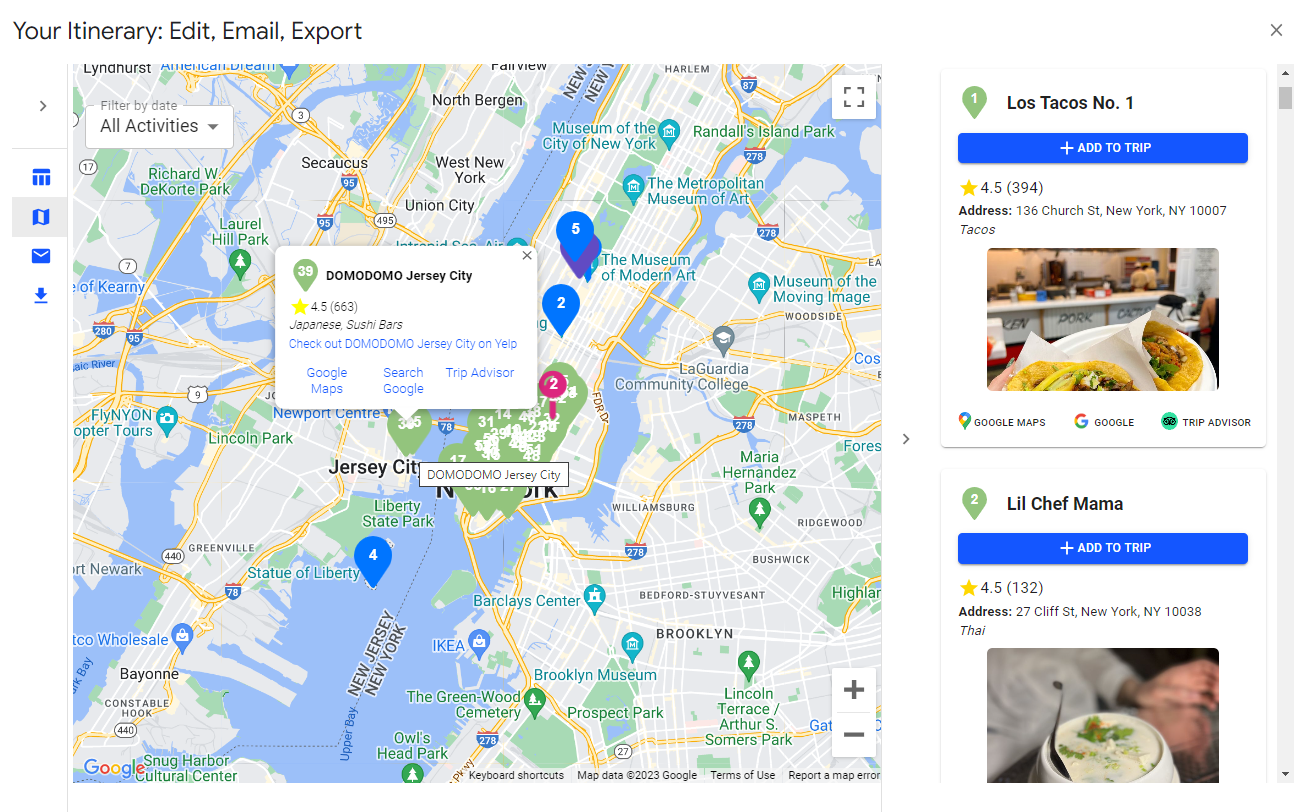This image is a screenshot of a driving trip map alongside additional navigation details. In the upper left-hand corner of the interface, there are options labeled "Your Itinerary," "Edit," "Email," and "Export." The primary focus of the image is a large map centered around the user's home, prominently displaying the D.O.M.O. Japanese Sushi Bar in Jersey City.

To the right of the map, there are trip suggestions and content details. The first suggestion lists "Location 1: Los Tacos No. 1" at 136 Church Street, New York, NY, with an option to add it to the trip. This location is notably far from the user's New Jersey starting point and seems irrelevant to the itinerary. Similarly, "Location 2: Little Chef Mama" at 27 Cliff Street, New York, NY, is suggested but is also impractically distant.

The map also shows local New Jersey towns such as Newport Center, Lincoln Park, Kearney, and Bayonne. These towns are much closer and more relevant to the user's location. The caption emphasizes the inaccuracy of the trip suggestions, noting that the system should recommend places within New Jersey, which offers many excellent taco options without crossing state lines.